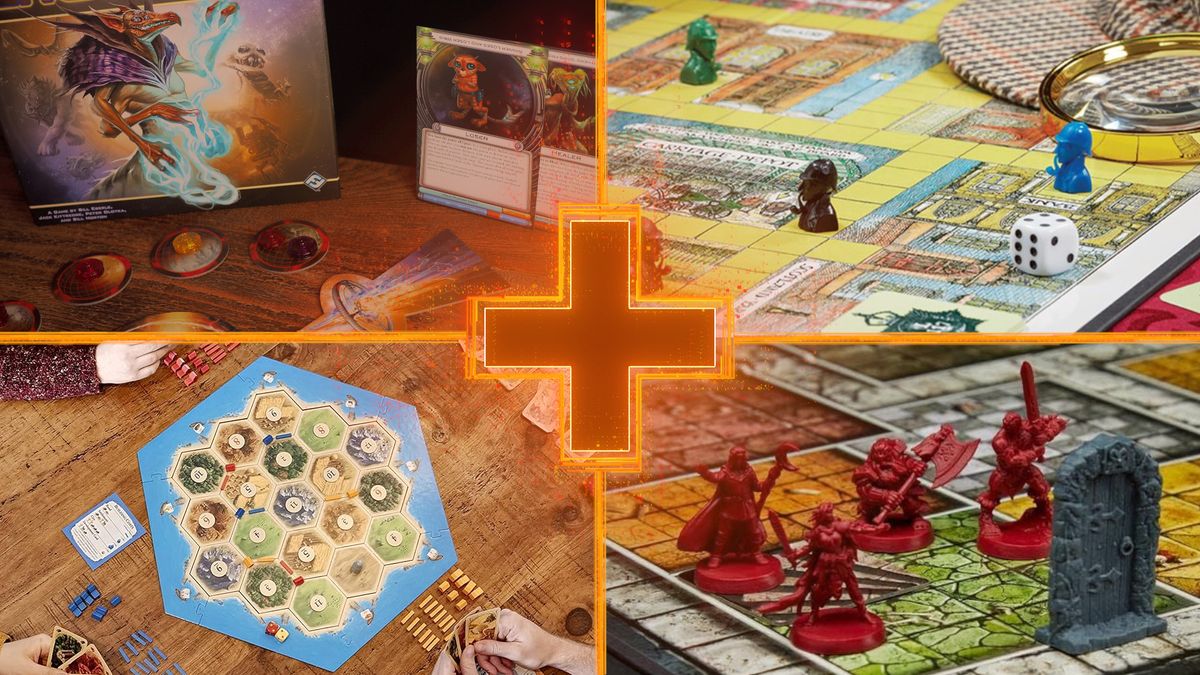The image consists of four separate panels arranged around a central brown cross with gold-edged corners. Each panel showcases a different board game. 

In the upper left, there's a game that features a cover image depicting a mythical creature that looks like a mix between a vulture and a dinosaur, surrounded by various smaller creatures. The game appears to involve cards, as several hands are seen holding them.

The upper right panel displays a board game with player pieces shaped like army soldiers, each with a distinctive look: a blue piece, a brown piece, and a green piece, all sporting either a cigar or tobacco pipe in their mouths. These are positioned on a board with yellow spaces, accompanied by a white and black die. There’s also a suggestion that the game might involve solving mysteries, as some pieces resemble Sherlock Holmes.

In the lower left, another board game is depicted, involving hexagonal tiles with numbers and colorful game pieces in yellow, blue, and red. Players' hands holding cards suggest that this game involves strategic card play.

The lower right panel shows a war-themed game, featuring red figurines of soldiers equipped with various medieval weapons like swords, axes, spears, and shields. These figurines are seen on a multicolored board that includes a distinctive gray medieval door, indicating a possible battlefield scenario.

Overall, the image captures the diverse and intricate nature of several board games, highlighting their unique pieces, colorful boards, and engaging themes.